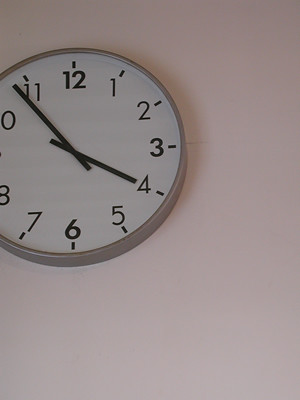The image captures a simple, round clock mounted on a wall, positioned towards the top left corner. The wall color oscillates between white and a light pinkish hue, giving a subtle yet distinct backdrop. The clock itself features a white face with black numbers; the 12, 3, 6, and 9 are bolded while the other numbers are in regular black font. The time displayed is approximately 4:54, with the hour hand on the 4 and the minute hand nearing the 11. The clock is slightly cut off, showing part of the number 8, missing the 9, and showing the zero on the 10. Its silver or grey outer frame adds a touch of contrast to the overall design, though it lacks any branding or minute marks that might offer additional detail. The image does not indicate any specific time of day.